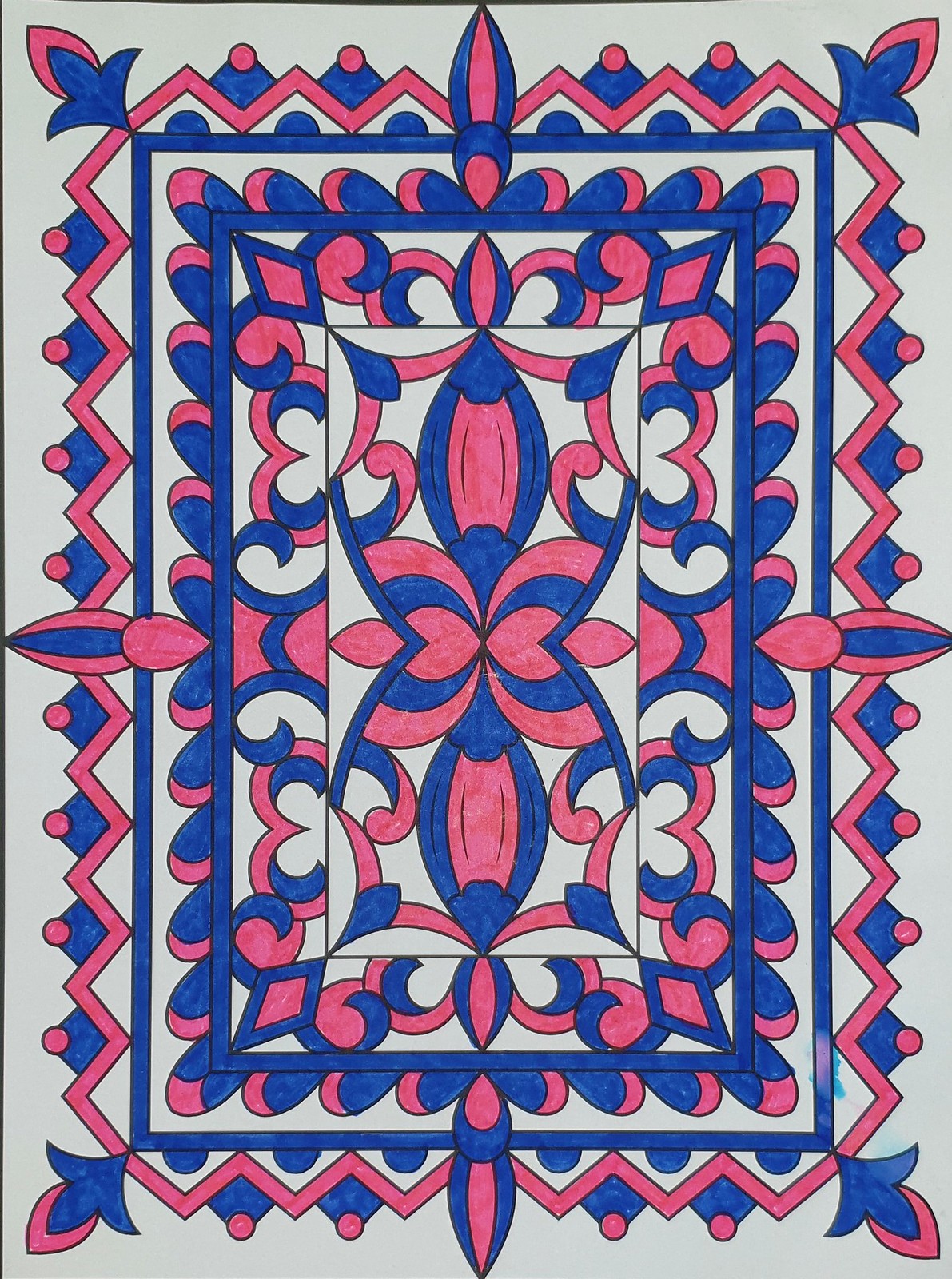This image showcases an ornate, vertically rectangular artwork, resembling the back of a traditional playing card and executed on a whitish-gray background. Created with felt markers, the dominant colors are dark blue and pink. 

The composition features multiple geometric shapes and borders. The outermost border consists of blue zigzag patterns with red dots nestled within each point. Inside this, a rectangular border displays ovals extending symmetrically at various angles. Moving inward, another rectangular border contains blue diamond shapes with red circles at their base, aligned in symmetry.

The corners of the artwork are adorned with flowery designs, resembling closed pink flowers with three petals or leaves. These floral motifs continue in the interior, complemented by large, petal-like blue and red figures, some extending from the bottom to the top and others from left to right, intersecting at the center. At the very core of the design is an intricate figure that combines butterfly wing-like shapes with an hourglass form, all colored in complementary shades of red and blue. Overall, the elaborate patterns and detailed borders create an impression of depth and complexity, making the piece appear almost rug-like.